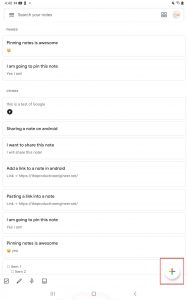A blurry screenshot of a mobile device displaying a typical user interface for an app or webpage. At the top, common phone icons are visible, though indistinct. Below, there is a shop icon and a search bar. Further down, there are sections with titles, each containing rectangular elements with text. Under one title, there are two rectangles with writing, and under another title, eight rectangular boxes each featuring a title and descriptions. The background is predominantly white. At the bottom, a navigation bar includes three icons: a three-lined menu icon on the left, an ambiguous house icon in the center, and an arrow pointing left on the right. Above the navigation bar, four smaller icons are situated towards the left. On the right side, a prominent red box contains a white circle with a rainbow-colored plus sign at its center.